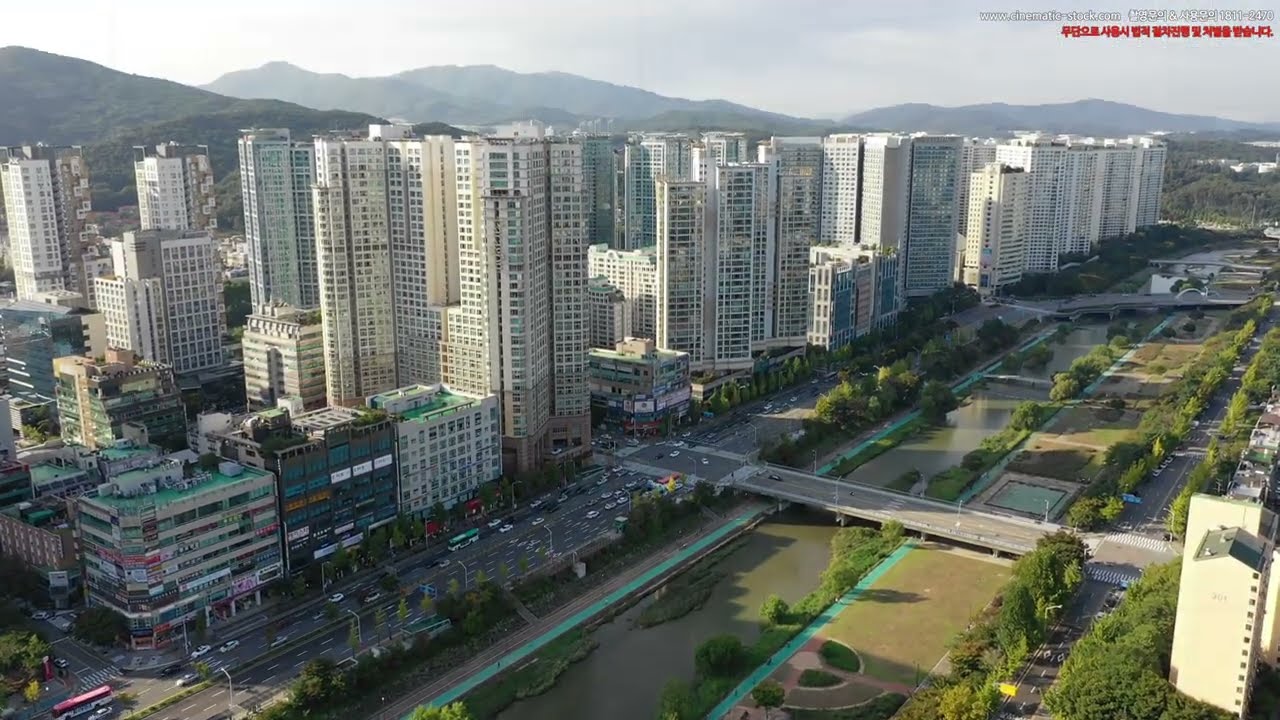The image presents an overhead view of a cityscape dominated by numerous, uniformly white skyscrapers on the left side. These high-rise buildings, characterized by their repetitive grids of windows and stories, stand adjacent to a major road that begins at the lower left corner and extends toward the upper right. This road intersects a verdant area featuring rows of trees and possibly a park or golf course. Just right below, there's a canal with a significant bridge crossing it, possibly accommodating up to four lanes of traffic, and at least two additional bridges are visible in the background. The scene extends further to reveal more skyscrapers, backed by towering mountains beneath an overcast sky. In the foreground, densely vegetated greenways and roads provide a stark contrast to the urban magnitude of the buildings. The vibrant, albeit cloudy, sky casts a somewhat gray light over the scene, enhancing the variety of colors present in this bustling cityscape. Notably, some red writing appears in the upper right corner of the image, though the specific lettering is unclear.